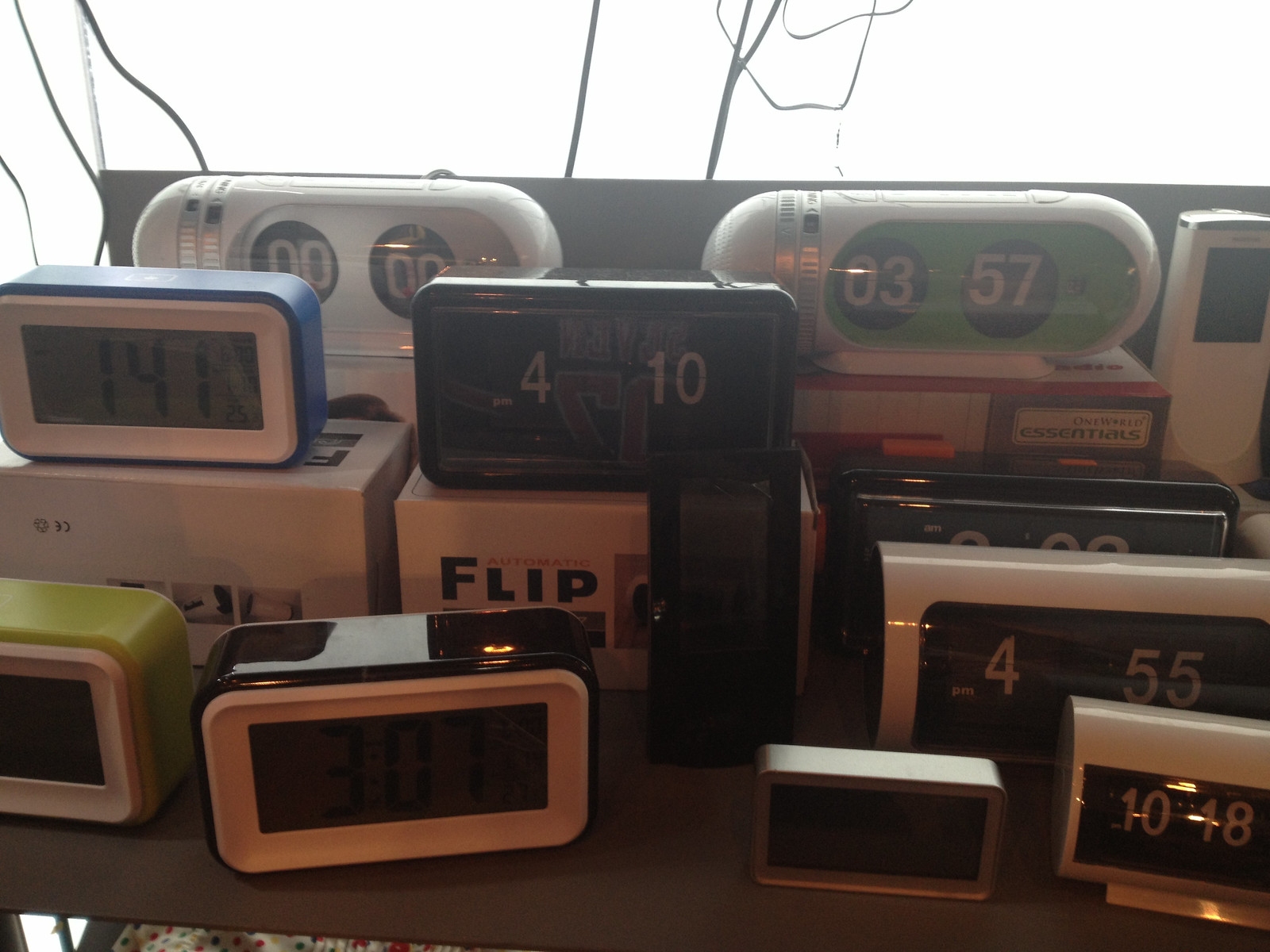This image presents a cluttered collection of various alarm clocks, arranged somewhat haphazardly on a light brown, potentially pressed-wood shelf. The scene appears to be in a store or second-hand shop given the vintage and diverse nature of the clocks. The shelf, taking up about 80% of the frame, is positioned against a backdrop that includes a bright window, casting a harsh white light and contrasting with the dimly lit interior where the clocks reside.

Starting from the bottom left, there is a lime green digital clock with a black screen outlined in white. Adjacent to it on the right is another similar-shaped clock in shiny black, displaying the time as 3:07. Behind the lime green one, there is a royal blue clock showing 1:41. At the very back, a white capsule-shaped clock with silver bands displays "00:00." To its right sits an identical capsule-shaped clock, but with a light green face showing the time 03:57.

In the middle of the image, a prominent all-black clock displays 4:10 in white digits, and to its right, another black clock is partially visible, obscuring its display. On the bottom right of the image, there are two cylindrical white clocks with black faces and white numbering; the larger one shows 4:55, while the smaller one reads 10:18.

The clocks are of varied shapes, colors, and designs, including at least one analog clock among the majority digital ones. Some clocks rest directly on the shelf, while others are stacked on small boxes, one of which is labeled "automatic flip." The detailed description of individual clocks suggests a mix of modern and retro styles, adding to the eclectic feel of the display.